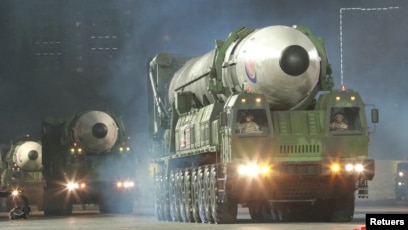The image depicts a nighttime scene of a military parade featuring three large, forest-green vehicles, each equipped with what appear to be white ballistic missiles mounted on top. The vehicles, which resemble a hybrid of tanks and heavy-duty trucks, are emitting substantial exhaust, creating a smoky atmosphere around them. Each vehicle has numerous wheels, with observers noting as many as nine or ten on each side. The vehicles' headlights illuminate the foggy or smoky surroundings, adding to the dramatic setting. The procession appears to be moving from the back towards the front right of the image. In the bottom right corner, the word "Reuters" is misspelled as "RETUERS." The scene is devoid of significant background details, though there are some lights that hint at structures or additional activity in the distance. This parade is likely a display of military strength, possibly coordinated by North Korea, showcasing their advanced weaponry and missile capabilities.